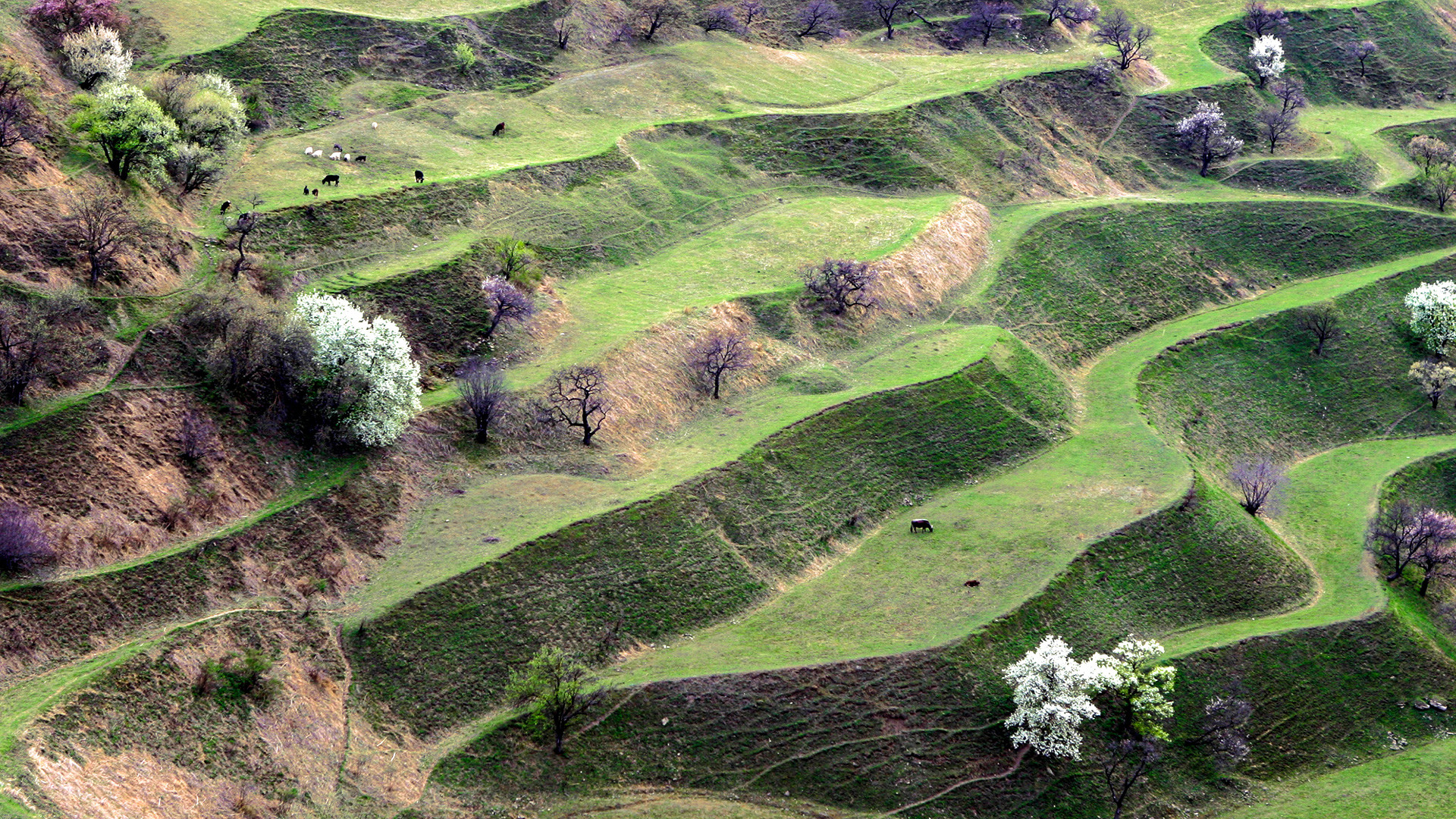The image depicts a vibrant and detailed painting of a terraced landscape, characterized by its vivid tiers of green grass that ascend like steps. The top left corner reveals earthy brown hills adorned with scattered flowers, transitioning to lush greenery towards the top right. Dominating the scene are various trees with purple leaves and others blanketed in white flowers. Across multiple platforms, you spot tiny animals, including black and white ones grazing. The middle of the painting features light green hilltops accented with white and yellow, alongside bushes in shades of blue and purple. The left side showcases dark brown cliffs with green vegetation, while the bottom right is populated by more white and purple trees. Throughout the piece, patches of darker green, brown stems, and branches add texture to the foliage. At the very top, a row of purple bushes with dark branches creates a striking contrast against the verdant backdrop.